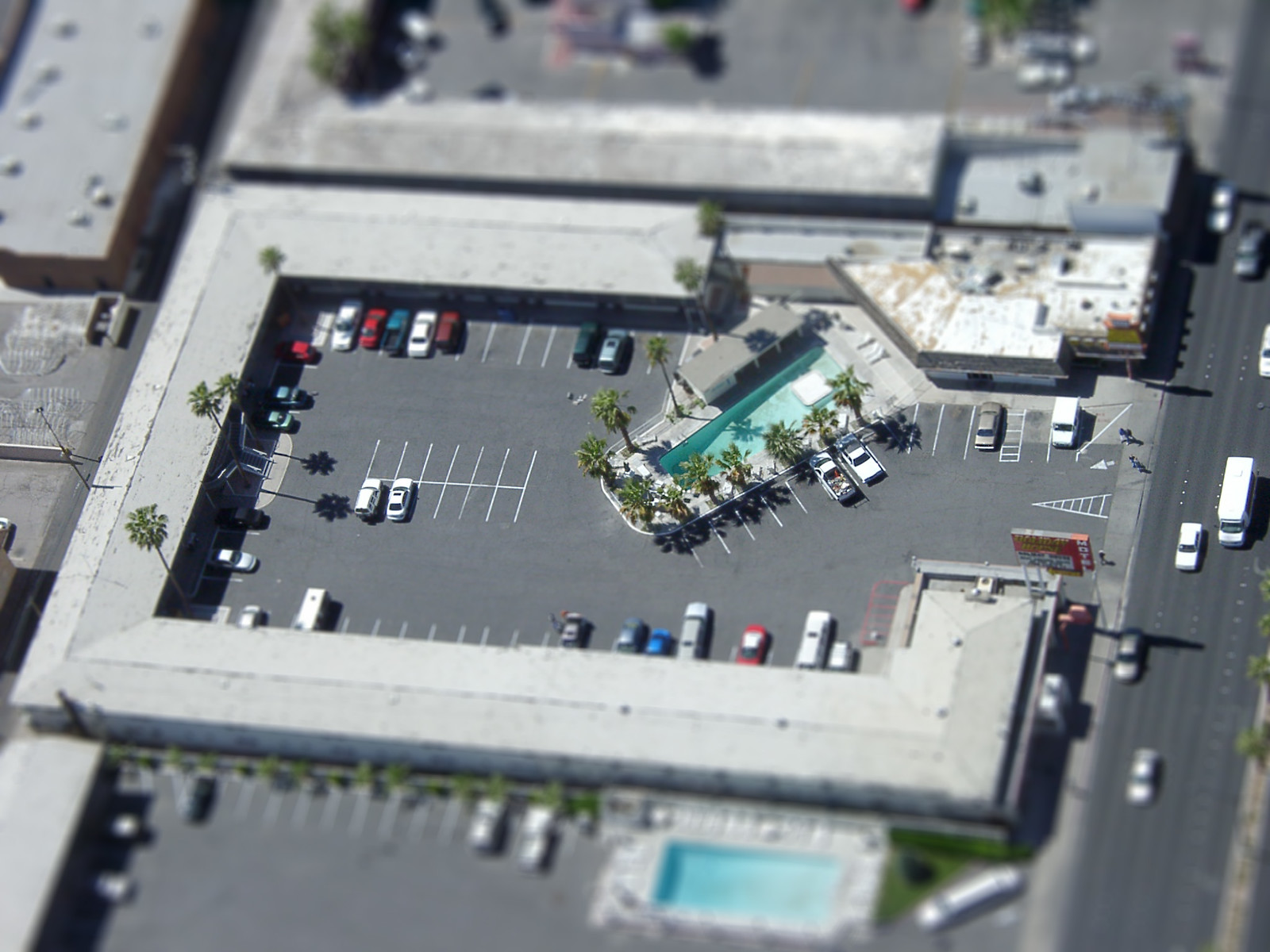The image is an aerial view of a detailed, photorealistic model depicting a hotel complex. The hotel, which has a hollow rectangular or G-shaped layout, encloses a central asphalt-covered parking lot with multiple delineated white lines for driving and parking spaces. To the right of the parking lot, a road with various toy cars, including a truck, provides access into the parking area. The building itself features a light gray roof and white exterior walls. In the center of the parking lot, a vibrant light blue swimming pool surrounded by lush green palm trees adds a touch of leisure to the scene. The palm trees are also scattered towards the back of the parking area, enhancing the model's detailed and lifelike appearance.